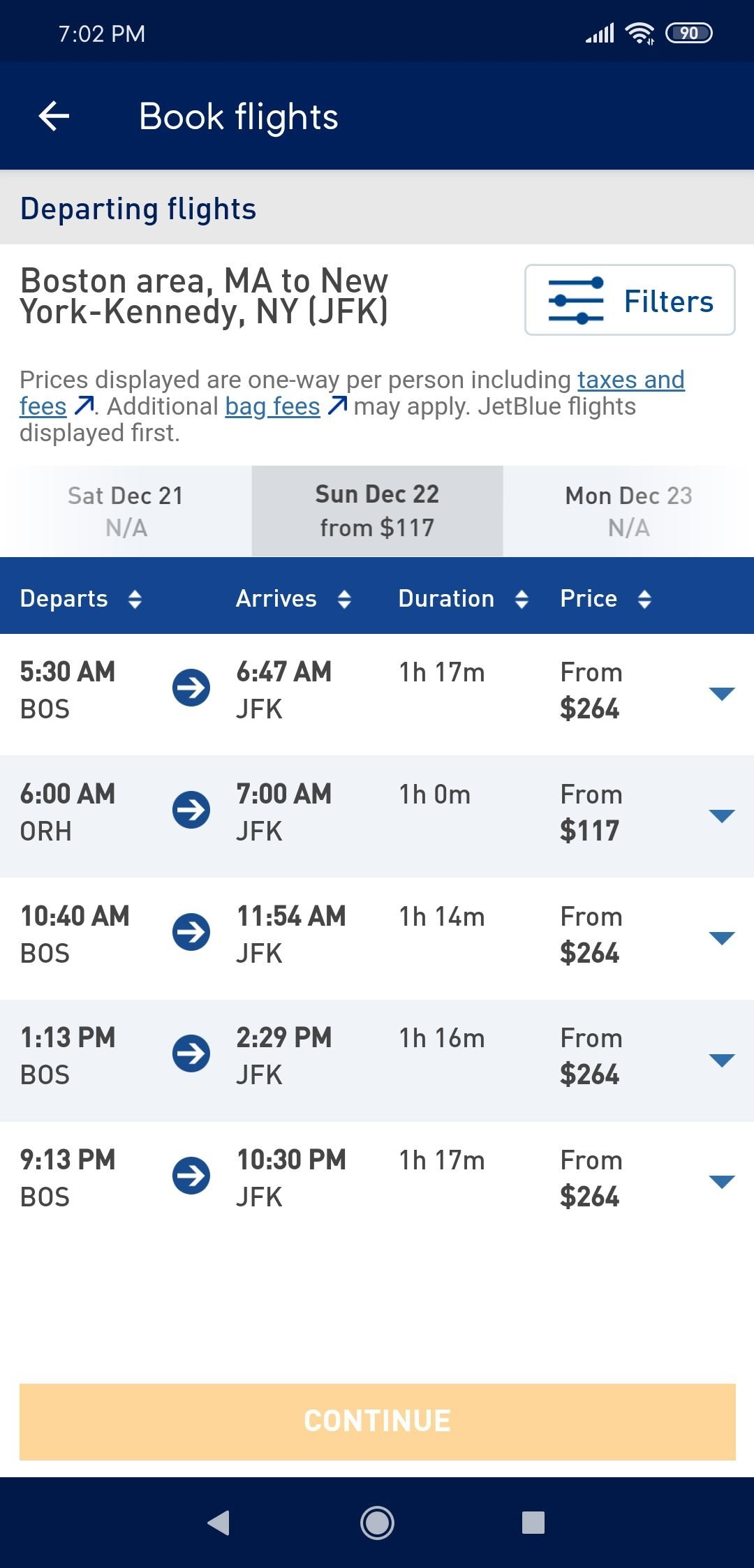The image depicts a digital interface for booking flights, likely captured from a smartphone or a computer screen at 7:02 p.m. The device displays 90% battery life. The header reads "Book Flights," followed by a section labeled "Departing Flights." The search details indicate flights from the Boston area, MA to New York, JFK. An array of filter options is available for refining the search. 

Below the header, a disclaimer states, "Prices displayed are one way per person including taxes and fees. Additional bag fees may apply. JetBlue flights displayed first." The available dates range from Saturday, December 21st, to Monday, December 23rd, with fares starting at $117. 

Detailed flight information is provided:

1. **5:30 a.m. (BOS) – 6:47 a.m. (JFK):** 1 hour and 17 minutes, starting from $264.
2. **6:00 a.m. (ORH) – 7:00 a.m. (JFK):** 1 hour, starting from $117.
3. **10:40 a.m. (BOS) – 11:54 a.m. (JFK):** 1 hour and 14 minutes, starting from $264.
4. **1:13 p.m. (BOS) – 2:29 p.m. (JFK):** 1 hour and 16 minutes, starting from $264.
5. **9:13 p.m. (BOS) – 10:30 p.m. (JFK):** 1 hour and 17 minutes, starting from $264.

At the bottom of the interface, there is an option to "Continue" with the booking process.